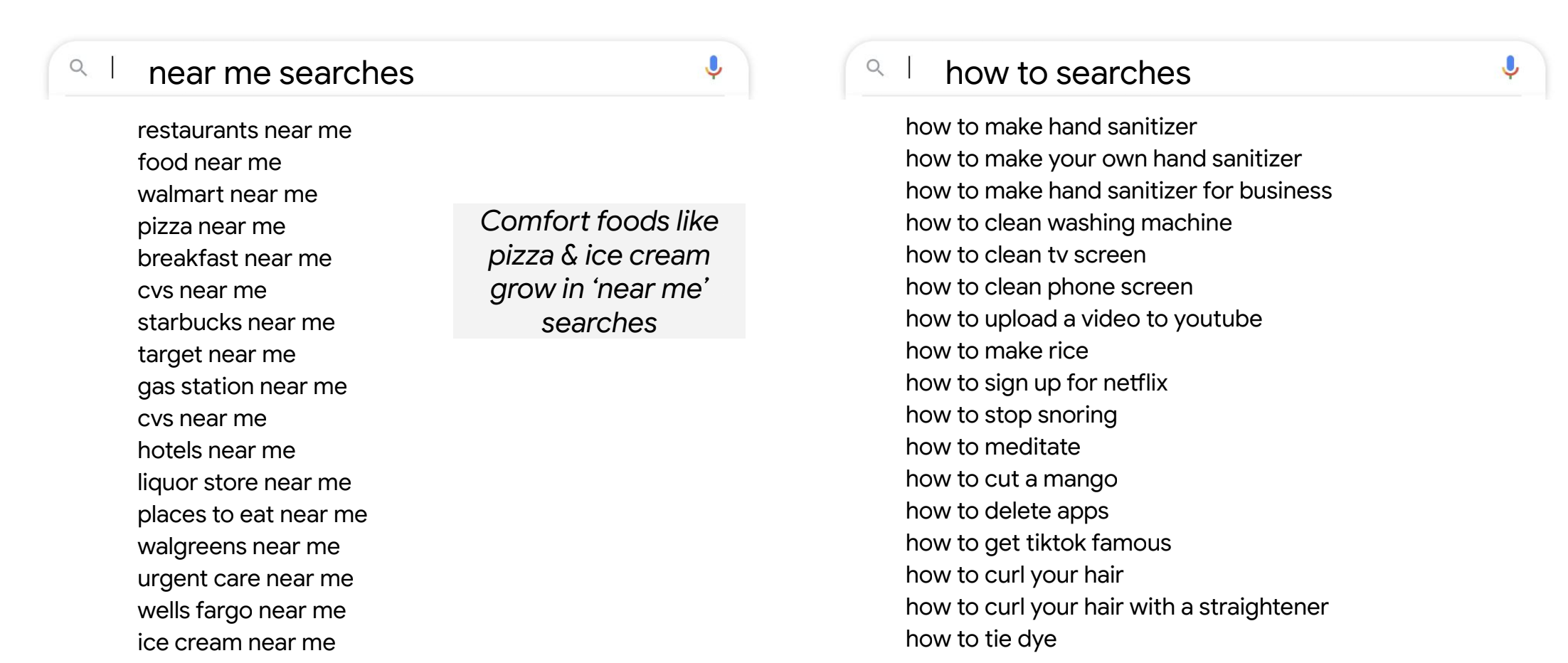The image portrays a white background with two prominent search bars and a compilation of popular search queries in black font. At the top of the image, a search bar showcases various "near me" searches. Listed below are search queries such as "restaurants near me," "food near me," "Walmart near me," "pizza near me," "breakfast near me," "CVS near me," "Starbucks near me," "Target near me," "gas station near me," "CVS near me," "hotels near me," "liquor stores near me," "places to eat near me," "Walgreens near me," "Urgent Care near me," "Wells Fargo near me," and "ice cream near me."

A small gray rectangle on the right side contains text that reads, "Comfort foods like pizza and ice cream grow in near me searches."

On the right side of the image, another search bar is visible, preceded by the text "how to" searches. Below this, a list of "how to" search queries includes "how to make sanitizer," "how to make your own hand sanitizer," "how to make sanitizer hand sanitizer for business," "how to clean," "how to clean a washing machine," "how to clean a TV screen," "how to clean a phone screen," "how to upload a video to YouTube," "how to make rice," "how to sign up for Netflix," "how to stop snoring," "how to meditate," "how to cut a mango," "how to delete apps," "how to use TikTok," "how to get TikTok famous," "how to curl your hair," "how to curl your hair with a straightener," and "how to tie-dye."